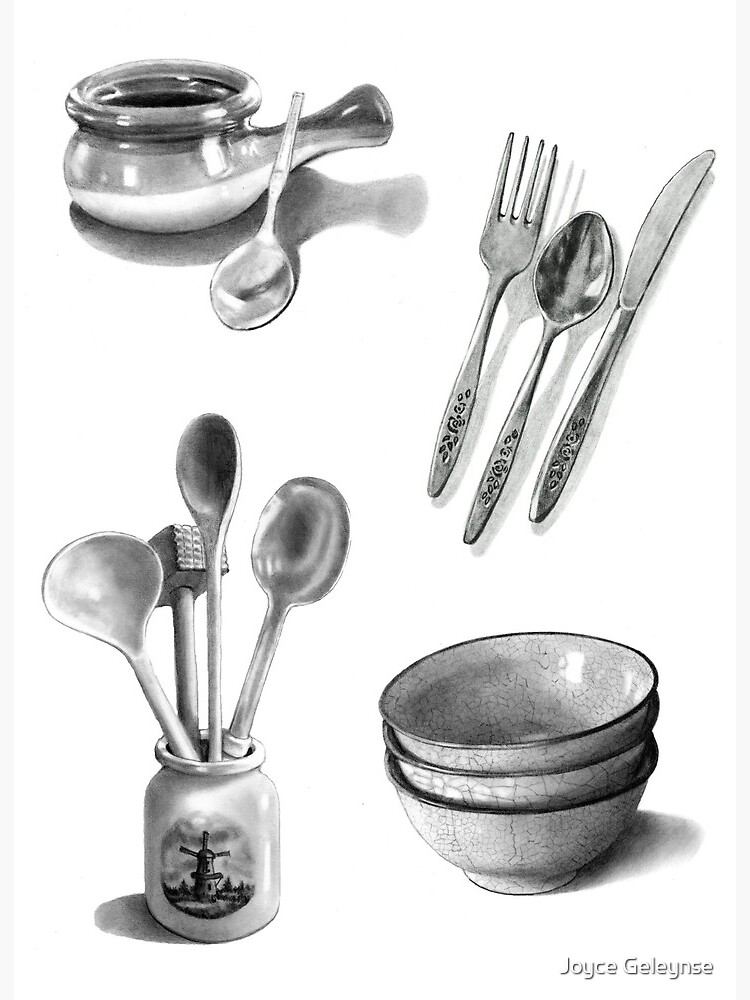The black and white illustration presents a collection of vintage kitchen items arranged in four distinct sections. In the top-left corner, there's a crock or sauce jar accompanied by a small spoon. Adjacent to this, in the top-right section, is a set of utensils including a fork, spoon, and butter knife with elegant handles. Moving to the lower-left section, a ceramic jar adorned with a Dutch windmill painting holds various large utensils such as a wooden spoon, a ladle, and a meat tenderizer. Finally, the lower-right section depicts a stack of three ceramic bowls, each appearing aged with visible cracks in the paint. The overall image highlights the nostalgic charm of these kitchen essentials set against a stark white background.